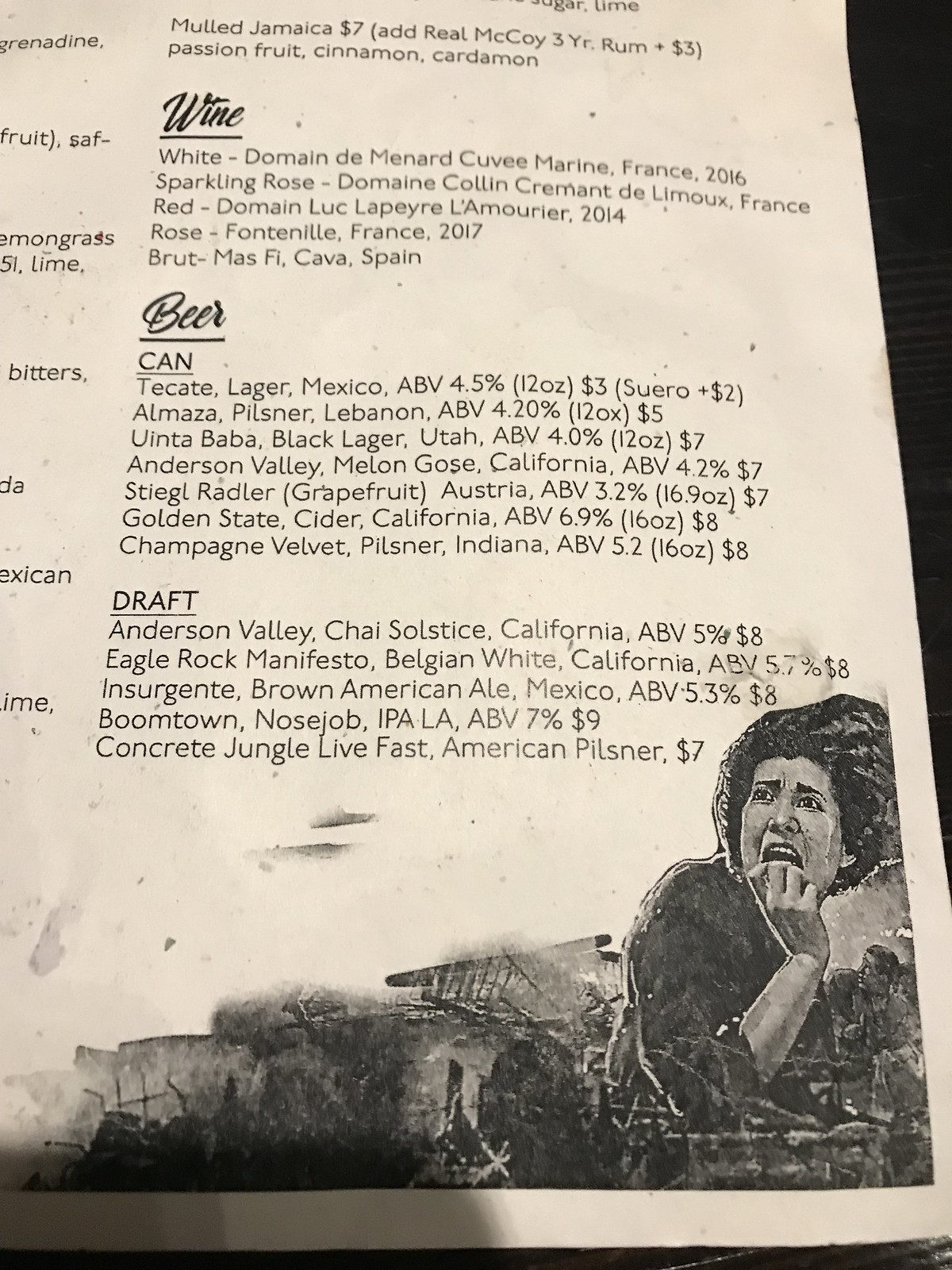A black table, possibly a desk, hosts a white paper-based menu. The bottom of the menu features an image of a distressed woman with her hand covering her mouth, likely set against a backdrop of a burning building. Above the image, the menu lists various types of wine: white, sparkling, rosé, red rosé, and brut. The wine section includes detailed options such as a "White Domaine de Menard, France 2016." For beers, the menu provides options for bottled and draft varieties, along with pricing. One featured beer is a "Tecate Lager, Mexico, ABV 4.5%, 12 ounces - $3.00," with a note in parentheses indicating "Suero + $2.00."